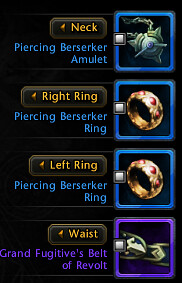The image appears to be a cropped screenshot from a video game, possibly World of Warcraft, depicting an equipment screen. On the right side, there are four square icons, each representing a different piece of equipment: a metal amulet, a pair of gold rings adorned with three red stones each, and a detailed blue and silver belt. To the left of these icons, there is a column listing the equipment slots and their corresponding items. The top slot, labeled in gold-yellow text, is "neck" with the item "Piercing Berserker Amulet." The next two slots, labeled "right ring" and "left ring," both show the "Piercing Berserker Ring" with identical images of a golden ring featuring three red jewels. The bottom slot, labeled "waist," displays "Grand Fugitive's Belt of Revolt" in a distinctive purple color, with an illustration of an ornate belt. The layout comprises two columns: item names and slots on the left, and corresponding images on the right, all set against a dark blue background.